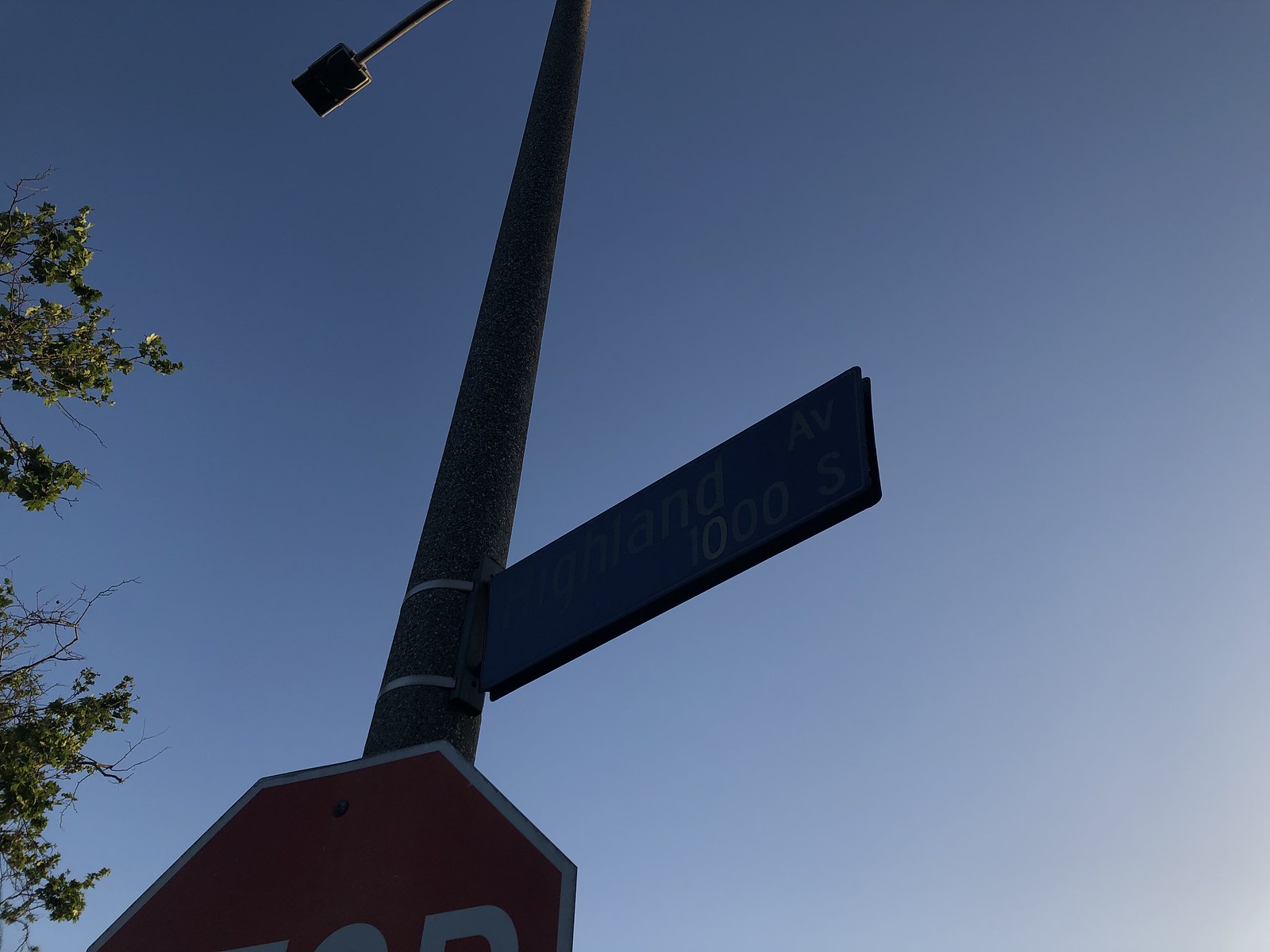The photograph captures a light pole viewed from the ground, looking upwards in the middle of a bright, clear day. Attached to the lower part of the pole is a stop sign, with only the top right corner visible, displaying the last letters "O" and "P." Above the stop sign, there are two metal straps securing a street sign that juts out to the right. This sign indicates the location as the 1000 block of South Holland Street with the inscription "Holland 1000 S." Ascending further, the pole extends at least 20 feet into the sky, curving to the left where a light fixture is affixed at its end. The light fixture remains off as it is daytime. On the left side of the image, the upper branches of a tree with lush green leaves are visible against the backdrop of a vivid blue sky. The sunlight, situated to the right, casts a bright glow, causing the objects in the photo to appear slightly silhouetted.